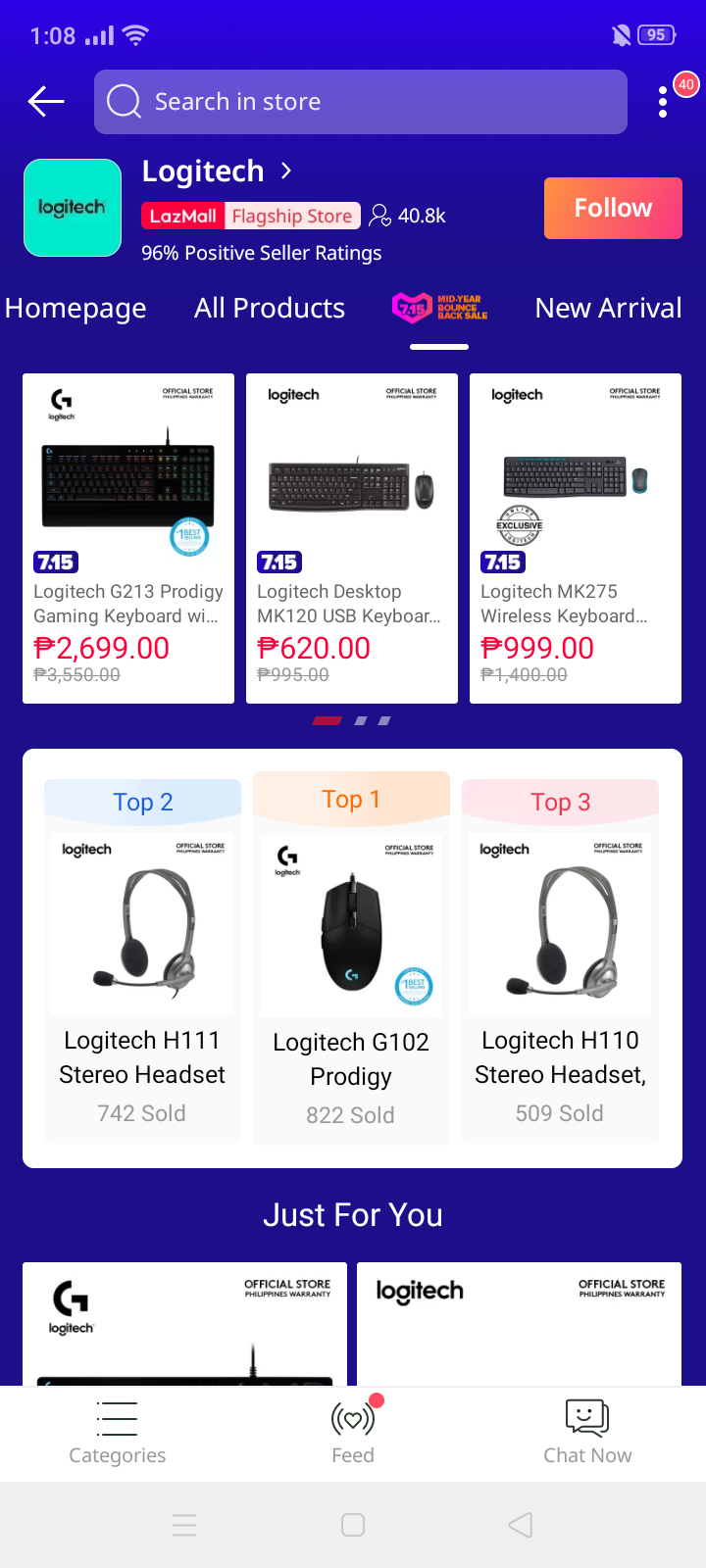Here's a cleaned-up and detailed descriptive caption for the image:

---

The webpage is a product page from Logitech's official website, designed with a darker blue background. At the top left corner of the screen, the phone's status bar displays the time as 1:08 PM, with full signal strength indicated for both data and WiFi connections. On the top right corner, an icon of a bell crossed out signifies that notifications are muted or the alarm is off. The battery indicator shows it is at 95%.

Central to the webpage is a search bar labeled "Search and Store" in white text. To the left of the search bar is a left-pointing arrow, while to the right are three dots with a red notification badge indicating 40 new updates.

The webpage header prominently features the Logitech logo within a blue box. It also highlights a "96% Positive Seller Ratings" badge and includes an orange "Follow" button positioned to the right. Below the header are navigation tabs labeled "Homepage," "All Products," an unreadable tab with a heart icon, and "New Arrivals."

The main content area showcases three different types of keyboards, each displayed within its own dedicated box along with their respective descriptions and prices. Below these, a large section named "Top Three Mice" ranks the top mouse products from right to left as "Top 2," "Top 1," and "Top 3," featuring two headsets and a mouse. At the bottom of the page, a segment labeled "Just For You" suggests additional personalized product recommendations.

---